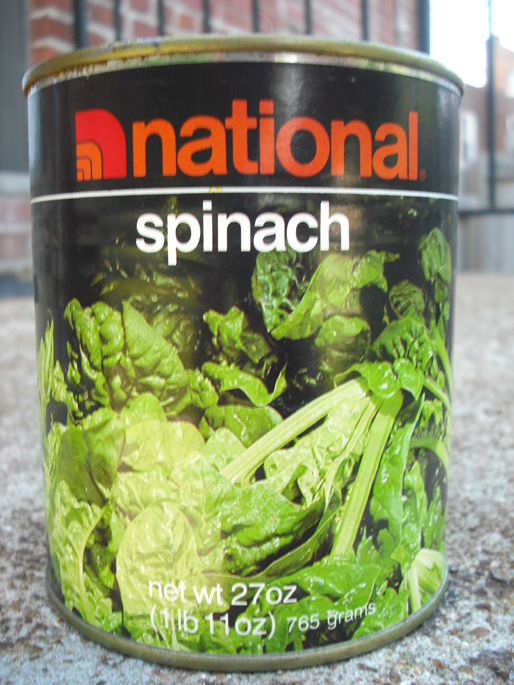This photograph captures a slightly weathered can of spinach with visible rust around its top edge, suggesting some age. The can is branded 'National,' with the brand name prominently displayed at the top in bold red block letters, flanked by an emblem comprising four arches—three orange and one red—on the left side. Below the brand name, a white line runs across the can, with the word 'Spinach' written in smaller white letters underneath. The can's label features an image of lush, green spinach leaves. Further down, the text indicates a net weight of 27 ounces (1 pound, 11 ounces or 765 grams). The can is placed on the ground, probably concrete, with a backdrop of a black gate and some buildings, possibly hinting at an outdoor setting.